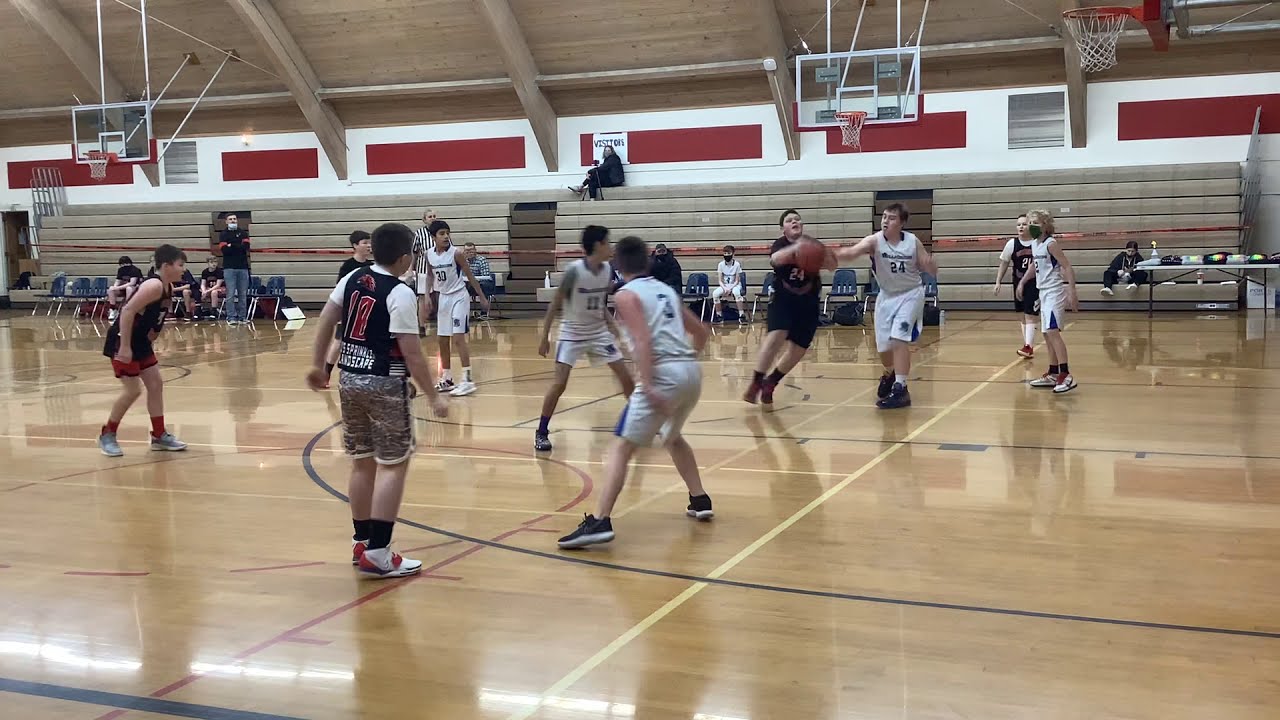This image features a youth indoor basketball game, with the players possibly being of middle school age. The court's shiny, buffed wood flooring stands out under the gymnasium lights. Two teams are competing: one in black jerseys with red text and the other in white jerseys with blue text, paired with white pants. One boy in black appears to be attempting a shot while navigating past an opponent, with a referee visible in the background overseeing the action. The background reveals an array of collapsed bleachers against a white wall accented with red, and a row of blue chairs in front of the bleachers where a few spectators or teammates are seated. Additionally, a person with a camera on a tripod can be seen atop the collapsed bleachers, likely capturing the game. Three basketball hoops are visible, one in active use and two against the wall in the background, adding to the gym's dynamic environment. The scene feels less like a highly attended game and more like a practice session or a scrimmage, given the minimal audience and the setup.